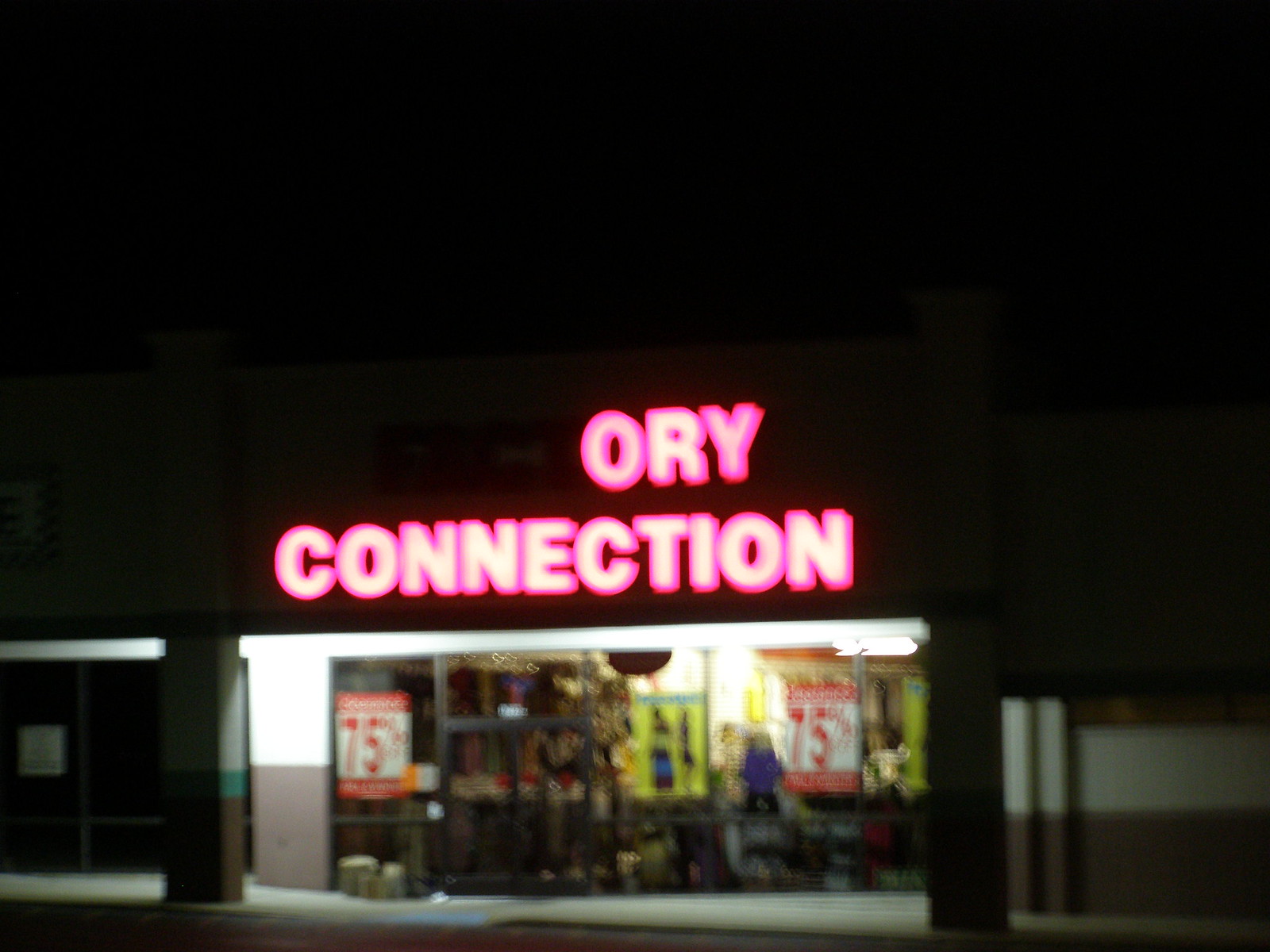A nighttime photograph captures the entrance of an enigmatic store. The top portion of the image is predominantly cloaked in darkness, while the lower third reveals an illuminated porch area, shedding faint light on the scene. The storefront features a set of double glass doors, flanked by brightly lit windows on either side. Positioned on the left and right side of the doors are prominent "75% Off" signs, hinting at a sale. Above the entrance, a bright pink neon sign partially stands out against a black background. The letters "O", "R", and "Y" are visible, with the word "Connection" glowing vividly beneath them. Inside the store, various items are dimly perceptible, though their exact nature remains unclear due to the photograph's blurriness.